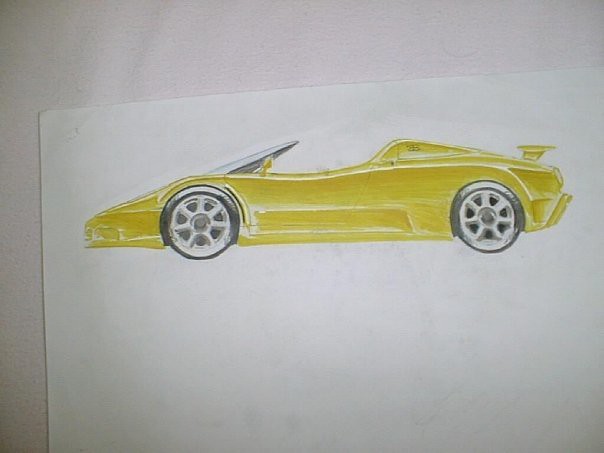This image captures a detailed sketch of a yellow sports car, specifically a convertible Lamborghini, drawn on the top left corner of a piece of white paper. The paper lies flat on an off-white or gray surface, with the visible area mainly showing the top portion of the sheet. The car is depicted from a side view, with the front facing left and the rear right. It features a sharply pointed front end and a small, prominent spoiler at the back. The windshield is sharply angled, offering minimal protection for the driver. The car’s tires are black and low-profile, accented with silver chrome wheels that exhibit gray and white highlights to create a reflective, shiny effect. The sketch uses a grayscale tonal range to emphasize the car's shadows and reflections, enhancing its three-dimensional appearance.